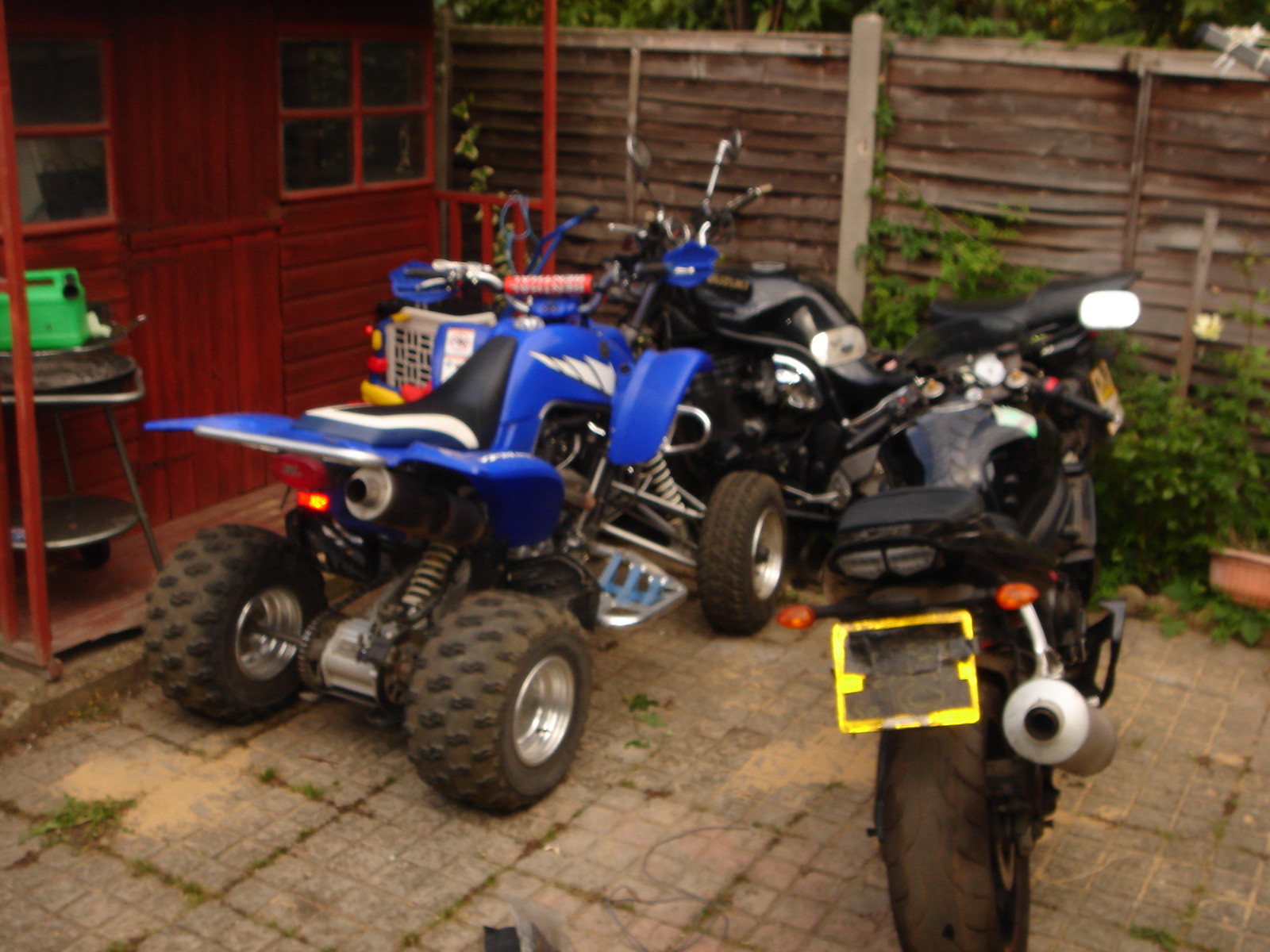This slightly blurry, low-resolution color photograph captures an outdoor scene dominated by three parked vehicles: a dark blue ATV with black wheels and a black seat, positioned on the left, and two black motorcycles arranged beside it. The ATV features notable black suspension with chrome accents near the engine and is parked on a concrete pad etched with smaller square patterns. To its immediate right, the first motorcycle boasts silver-outlined handlebars and circular mirrors, while the second motorcycle, furthest right, displays rectangular mirrors with rounded corners and a large silver muffler extending from its right side. This rightmost motorcycle’s yellow license plate is obscured by black electrical tape. Completing the scene, a small shack made of maroon wood lies to the left of the ATV, showcasing a maroon door and windows adorned with maroon crossbeams. Nearby, a lime green gas can sits atop a two-tiered steel stand with bent legs. In the foreground, a light gray wooden fence with a mix of light and dark brown cross beams defines the boundary of this cobblestone-like patio area.